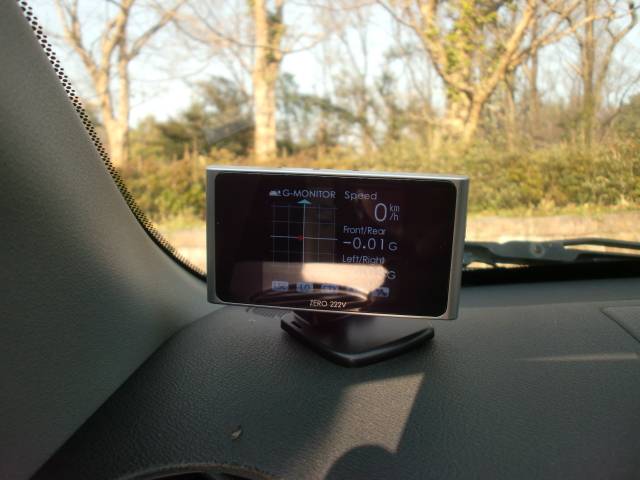This photograph captures a detailed view of the interior of a car, focusing primarily on the dashboard. The image highlights the left corner of the dashboard, where a mounted monitor labeled "G Monitor" is prominently displayed. This monitor provides various readings, including speed, front and rear calibration, and a left front calibration, all depicted in white font along the bottom of the screen. The display also features a graph with a vertical and horizontal axis; the vertical line culminates in a blue arrow tip, and a red dot is positioned at the center of the graph, which is set against a lighter grid backdrop.

A reflection, likely caused by sunlight streaming in from the left, is visible on the glossy surface of the monitor's screen. The monitor itself is encased in a gray frame and mounted on a black pedestal. Just behind the monitor, a windshield wiper is partially visible, hinting at the car's exterior. 

Through the windshield, a serene landscape of light-colored bark trees and some foliage can be observed, suggesting an early spring setting. The absence of fallen leaves and the presence of greenery reinforce this seasonal suggestion. The sky is a clear, light blue with no visible clouds, indicating a sunny day.

The car's interior features a black dashboard and light gray side walls, creating a sharp contrast that adds to the overall composition. This well-lit and vibrant image effectively combines technological sophistication with natural beauty.